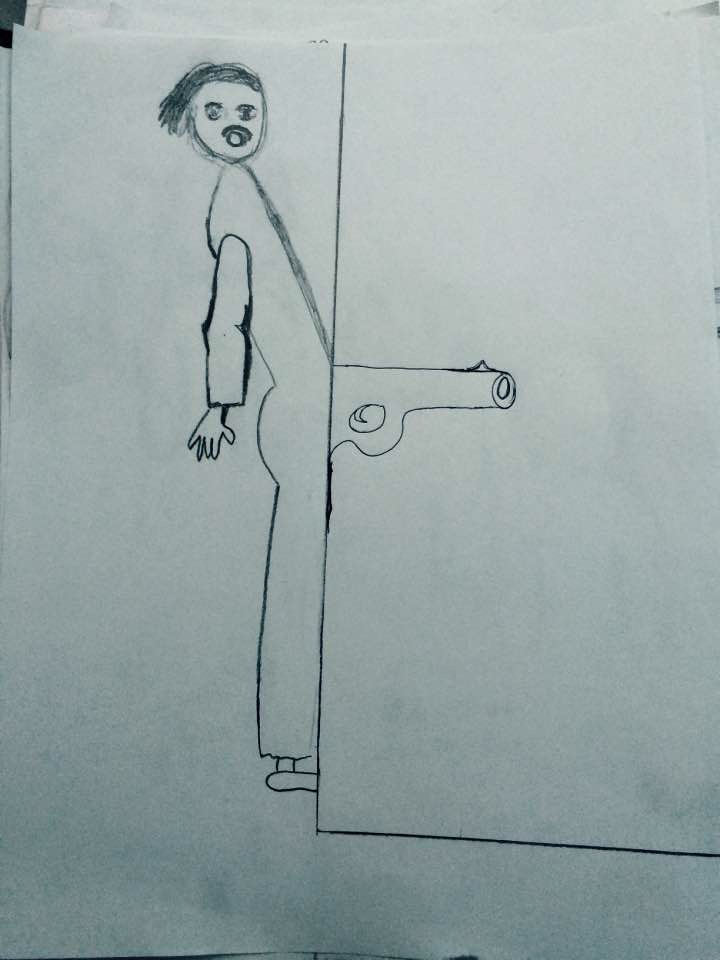The image is a humorous drawing depicting a man with slicked-back hair and a mustache, seemingly drawn in black pen or pencil on a slightly dirty white sheet of paper, with other papers visible underneath. The man is positioned at the edge of a wall, with only his legs, body, arms, and face visible, while his pelvic area is obscured behind the wall. Intriguingly, at the point where his pelvic region would be, a gun's barrel is drawn on the wall, creating the illusion that the man’s anatomy is replaced by the gun. The drawing style and context suggest it might have been created by a younger artist, adding to its crude and comedic nature.